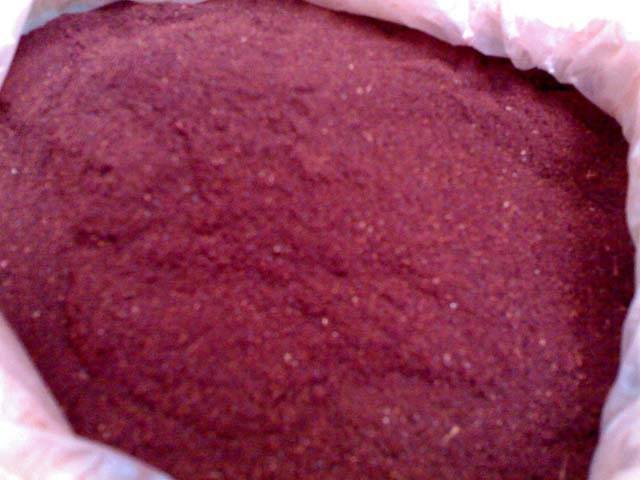The image is a horizontal, rectangular close-up of a dark red, irregularly shaped object that is possibly a dense pile of sandy material or a loaf of bread. The object features a predominantly dark red color with specks of brighter, tan-like shades and metallic sparkles distributed throughout. The material or object appears to form a mound, with the highest point located near the top left corner of the image. The entire scene is encased in a white plastic bag, which surrounds most of the image except for the far upper right corner where sunlight streams down, illuminating the bag. The background at the very corners showcases a pink, blue, and white abstract patterned fabric.